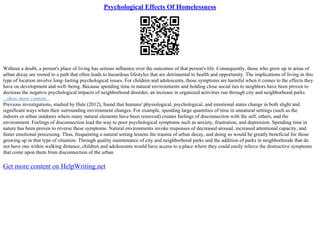The image is a close-up of a white background document, possibly a page from a book or flyer. At the top, there is a dark blue, underlined title that reads "Psychological Effects of Homelessness." Directly beneath this title, there is a square QR code. At the bottom of the image, another dark blue, underlined hyperlink text states "Get more content on helpwriting.net." The document contains two paragraphs of black text that are too small to read clearly. Within these paragraphs, there is an additional blue hyperlink, but it is also too small to decipher. The QR code is described as being fuzzy, similar to a TV screen, with four small squares—three have an interior black section with white and black borders, while the one in the far-right corner is notably smaller.